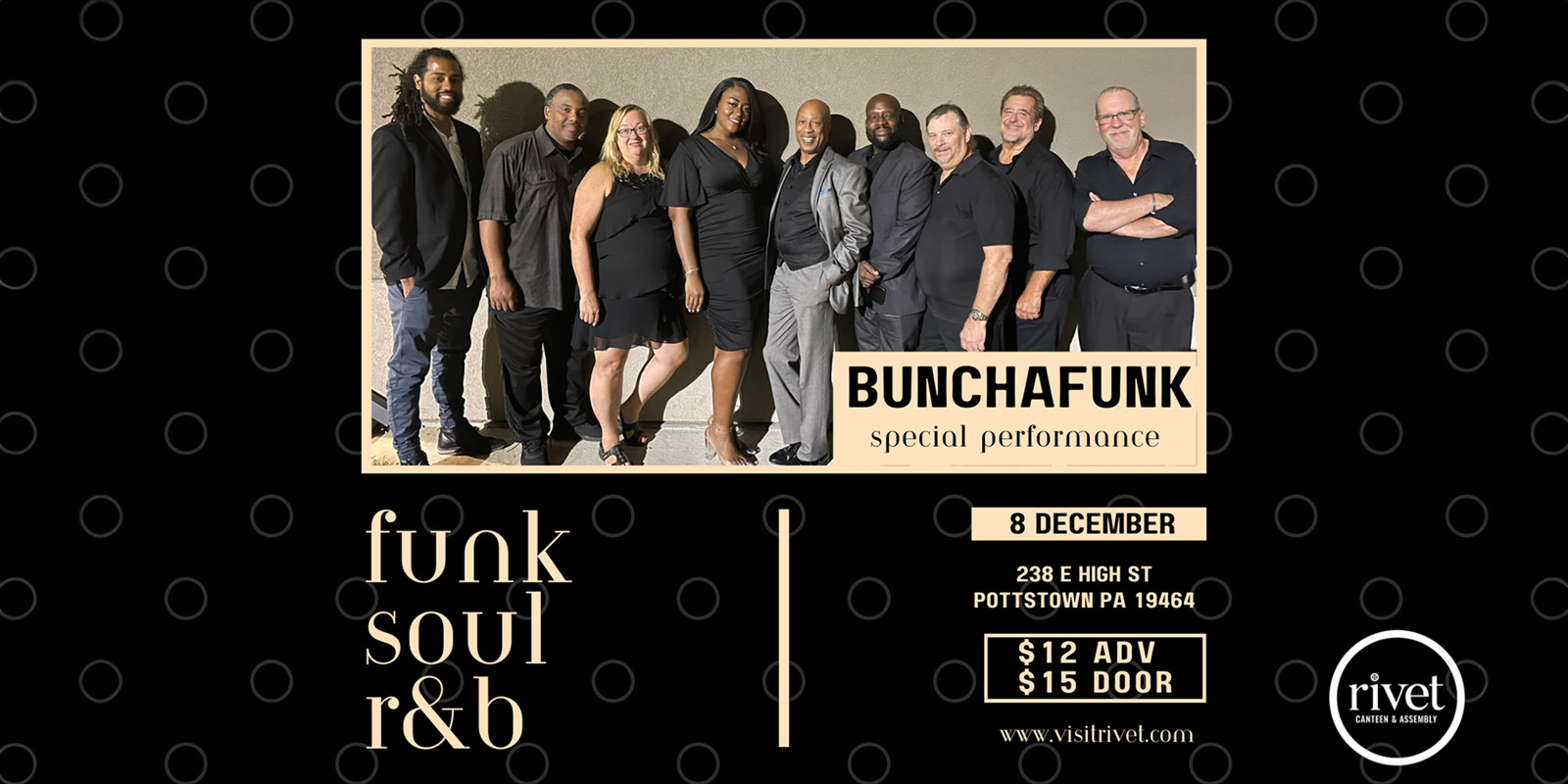This concert poster, sponsored by Rivet, promotes a special performance by the band Buncha Funk. The poster features a simple yet striking black background adorned with small gray circles and sporadic yellow line circles. The central image, occupying half of the space, showcases the nine-member band, which includes seven men and two women (one black and one white). The band members are dressed in predominantly black attire, with the central figure being a bald black man in a light gray suit. They perform a mix of Funk, Soul, and R&B music.

Positioned on the left below the image, the genres "Funk, Soul, R&B" are highlighted, whereas the right side notes the performance details. The concert is set for December 8th at 238 East High Street, Pottstown, Pennsylvania, 19464. Ticket prices are $12 in advance and $15 at the door. Additional information can be found on the venue’s website, www.visitrivet.com. The text throughout the poster is primarily a light yellowish-orange color. Finally, Rivet Canteen and Assembly's branding is visible in the bottom right corner, emphasizing their role in the event.